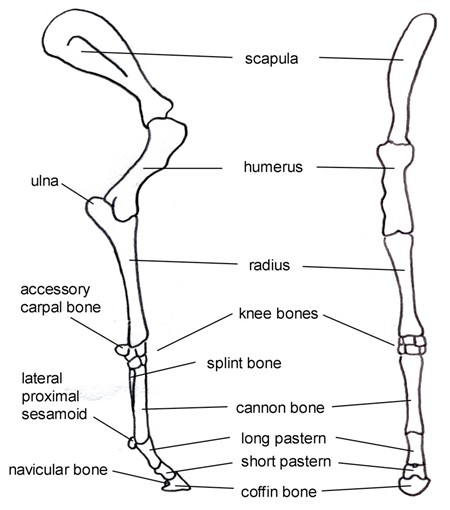The illustration depicts the skeletal structure of what appears to be a horse's leg, presented in a detailed, educational format akin to what might be found in a biology textbook. The image is divided into two views: the left side presents a side profile of the leg facing to the right, while the right side shows a frontal view. Both views share a white background with faint horizontal and vertical gray lines, measuring approximately four inches high and three inches wide.

In the center between the two leg views, black lines extend outward to label various bones from the top down, beginning with the scapula. The next labeled bone is the humerus, followed by the radius, knee bones, cannon bone, long pastern, short pastern, and finally the coffin bone at the bottom.

Additional labels are positioned to the left of the side profile view, identifying the ulna at the top, accessory carpal bone near the knee, splint bone below that, lateral proximal sesamoid further down, and the navicular bone at the back of the hoof. The detailed labeling and multiple perspectives provide a comprehensive understanding of the horse's leg skeletal anatomy.